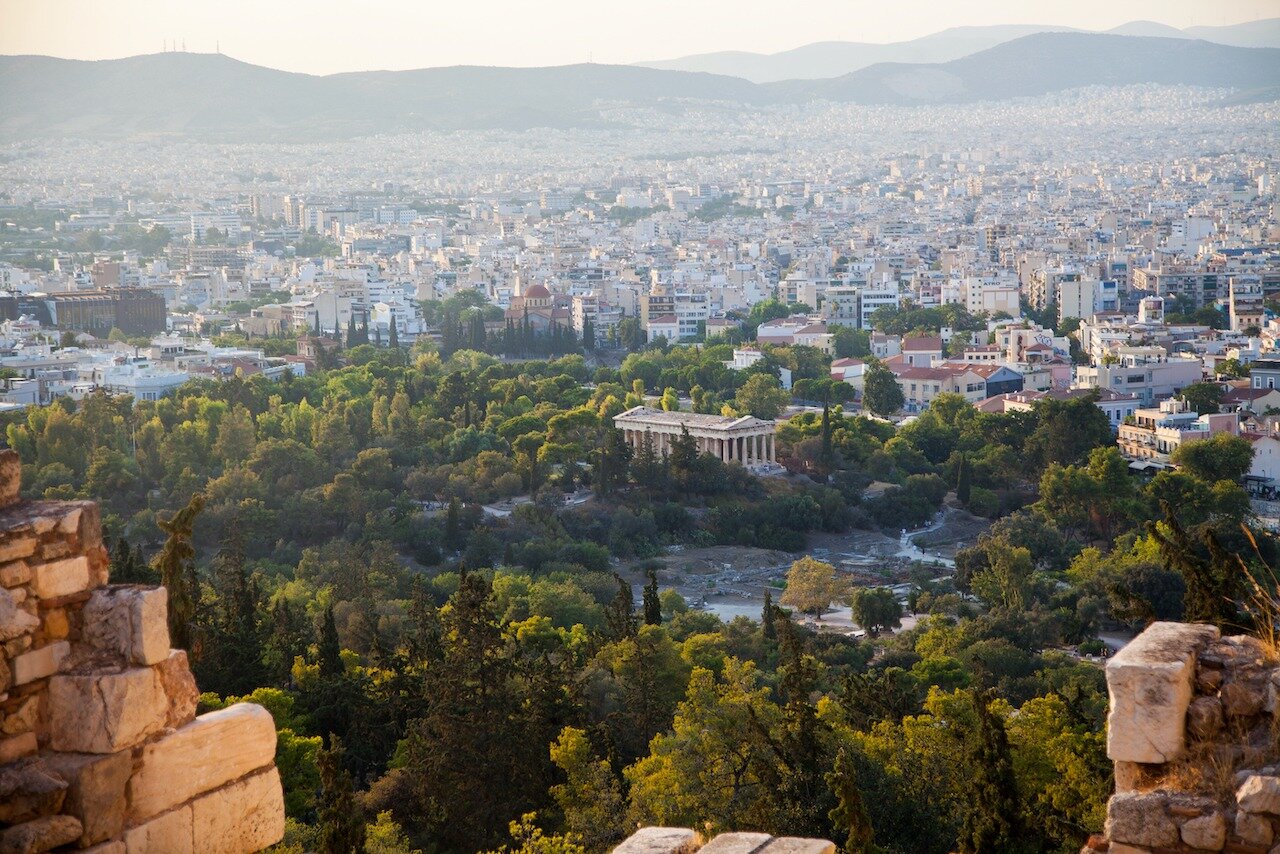The image captures a stunning and detailed view from an elevated ancient ruin, possibly Greece, overlooking a complex landscape. In the immediate foreground, remnants of a stone wall or building are visible, anchoring the perspective. Just beyond, a patch of white pathways winds through a park that is rich with green trees and ancient ruins, including a prominent Greek temple resembling the Parthenon at the center. This temple is surrounded by lush greenery, suggesting a necropolis or historical area, where people can be seen meandering through the park. 

Beyond this historic site lies an expansive, densely populated urban city, characterized by countless white buildings and towering skyscrapers, extending as far as the eye can see. Further in the distance, the cityscape transitions into dark and light gray hills, capped by a hazy, light gray sky. The sun, low on the horizon, casts a soft light across the entire scene, indicating that it might be either early morning or late evening. The overall composition merges ancient history with modernity, framed by natural elements and ambient light.